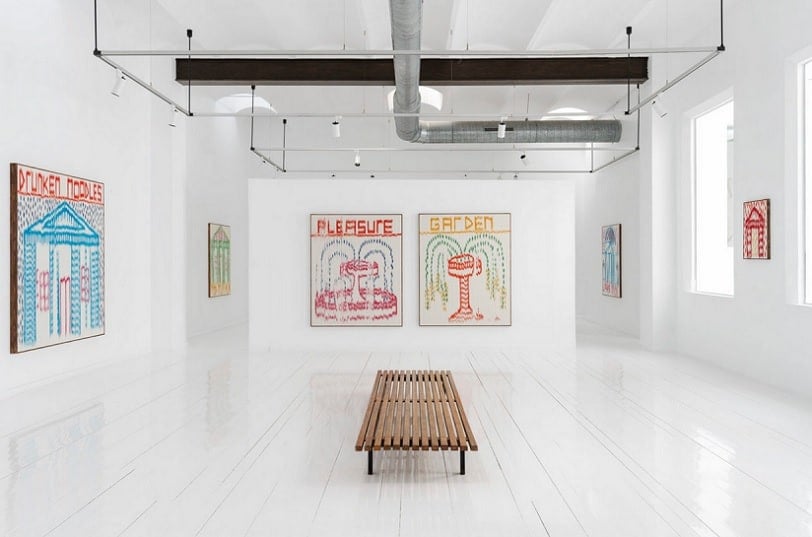This 3D color illustration, likely created using an app like SketchUp, captures the interior of a modern, minimalist gallery or museum space. The point of view looks downward at a low, wooden slat bench placed centrally on a white, painted wooden floor. The room’s walls and ceiling are stark white, adorned with industrial piping and mounted lights on a metal framework.

In the foreground, at the center bottom, the wooden bench stands out against the pristine background. Directly ahead, on the far wall, are two prominent art pieces. The left artwork displays the word "Pleasure" in red, with an illustration of a fountain in vivid red and blue. Beside it, the word "Garden" is depicted in yellow above another fountain design incorporating red, green, and blue simple shapes.

On the left wall, the most noticeable artwork resembles the facade of a blue pillared building with the words "Drunken Noodles" inscribed in red over it. Further down, additional artworks are hung, though their details are less discernible due to the viewing angle. On the right wall, paintings also hang, with light streaming through windows to the far right enhancing the display space.

Overhead, there's a complex network of silver venting and metal piping, with scaffolding and interior lighting illuminating the gallery. Beyond the main wall holding the "Pleasure" and "Garden" pieces, the room extends further, revealing more walking areas and additional art, emphasizing the space's function as an art exhibit.